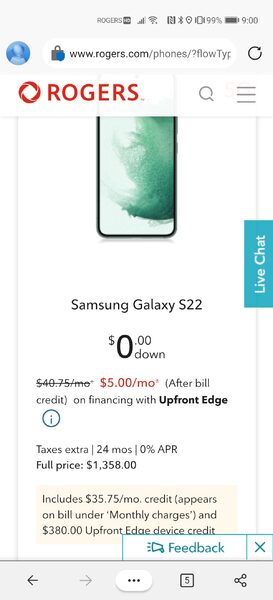The image depicts a smartphone screen displaying a web page. At the very top, the screen shows standard status indicators, including the time set to 9:00, battery percentage, and a Bluetooth signal icon. The browser's address bar features a lock icon beside a blue circle, indicating a secure connection, followed by the URL "www.rogers.com/flows" and additional text.

Directly below the address bar, the page prominently displays the Rogers logo in red letters, accompanied by a red circular icon. There is a search button near this header. The main content area showcases a promotional offer for a Samsung Galaxy S22 smartphone. The display features a green wallpaper on the phone's screen and highlights an enticing deal: "$0 down" with a reduced monthly payment of $5 instead of the usual $40.75, thanks to bill credits. The financing terms indicate zero APR over 24 months, culminating in a total cost of $1,358. This figure includes a $35.75 monthly credit applied to the bill and a $380 Upfront Edge device credit. Additional text notes that taxes are extra.

At the bottom of the screen, several navigation buttons are visible: a back arrow, a forward arrow, a button with three dots, a tab box currently showing the number 5, and an icon resembling a hairpin. The overall page design features a predominantly white background with black text, highlighted by various colors and logos to attract attention to specific details.